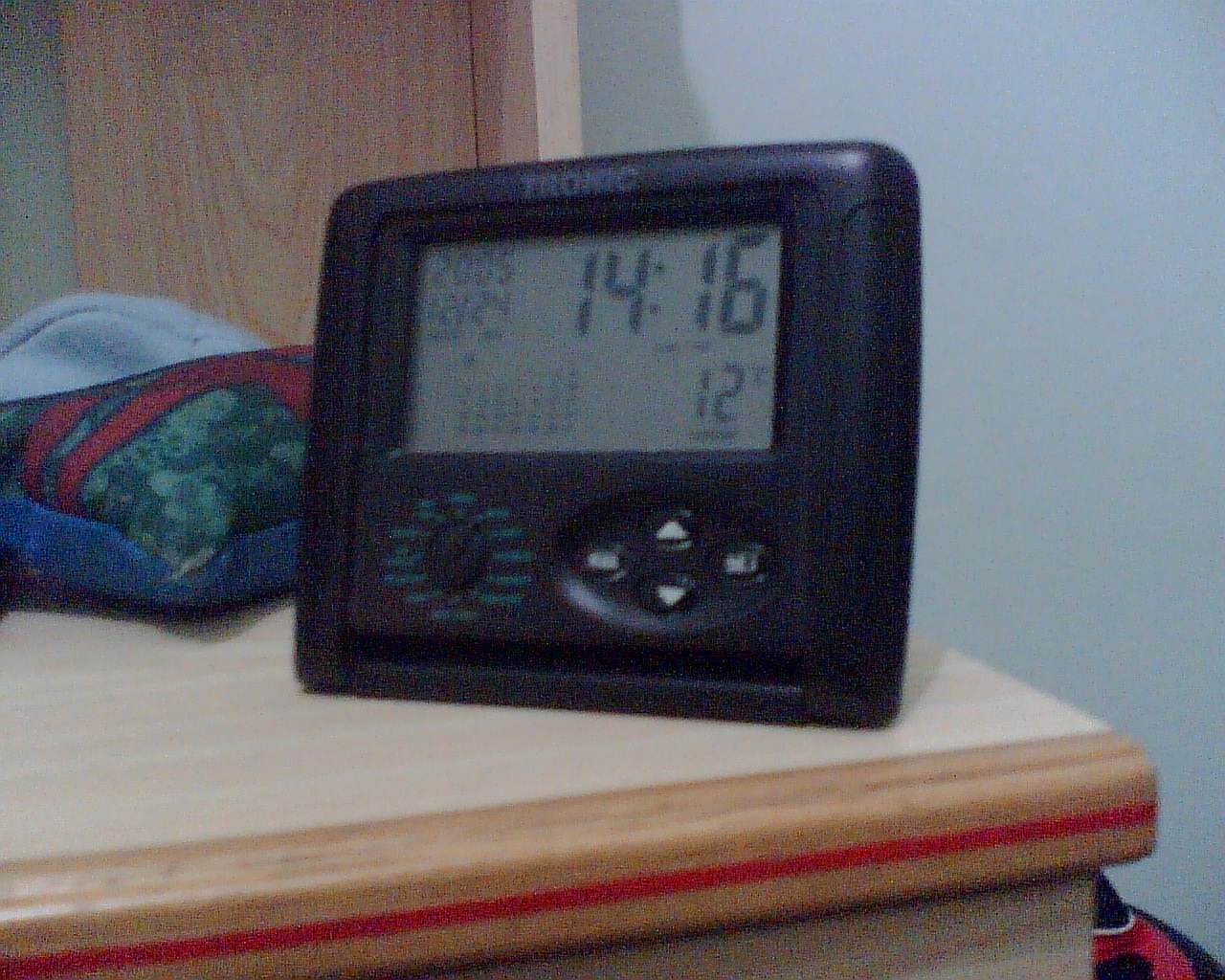This grainy photograph depicts a digital clock, likely from a brand called Tronic, situated on a nightstand. Despite the blurriness, the clock’s digital display prominently shows the time as 14:16. Beneath the display, circular up and down arrows are visible, accompanied by several other indistinct buttons. To the left of the display, there is a black dial equipped with a small arrow. The digital display also indicates the date as 2005-12-24. The nightstand, made of bleached wood, serves as the clock’s resting place in what appears to be a corner of the room.